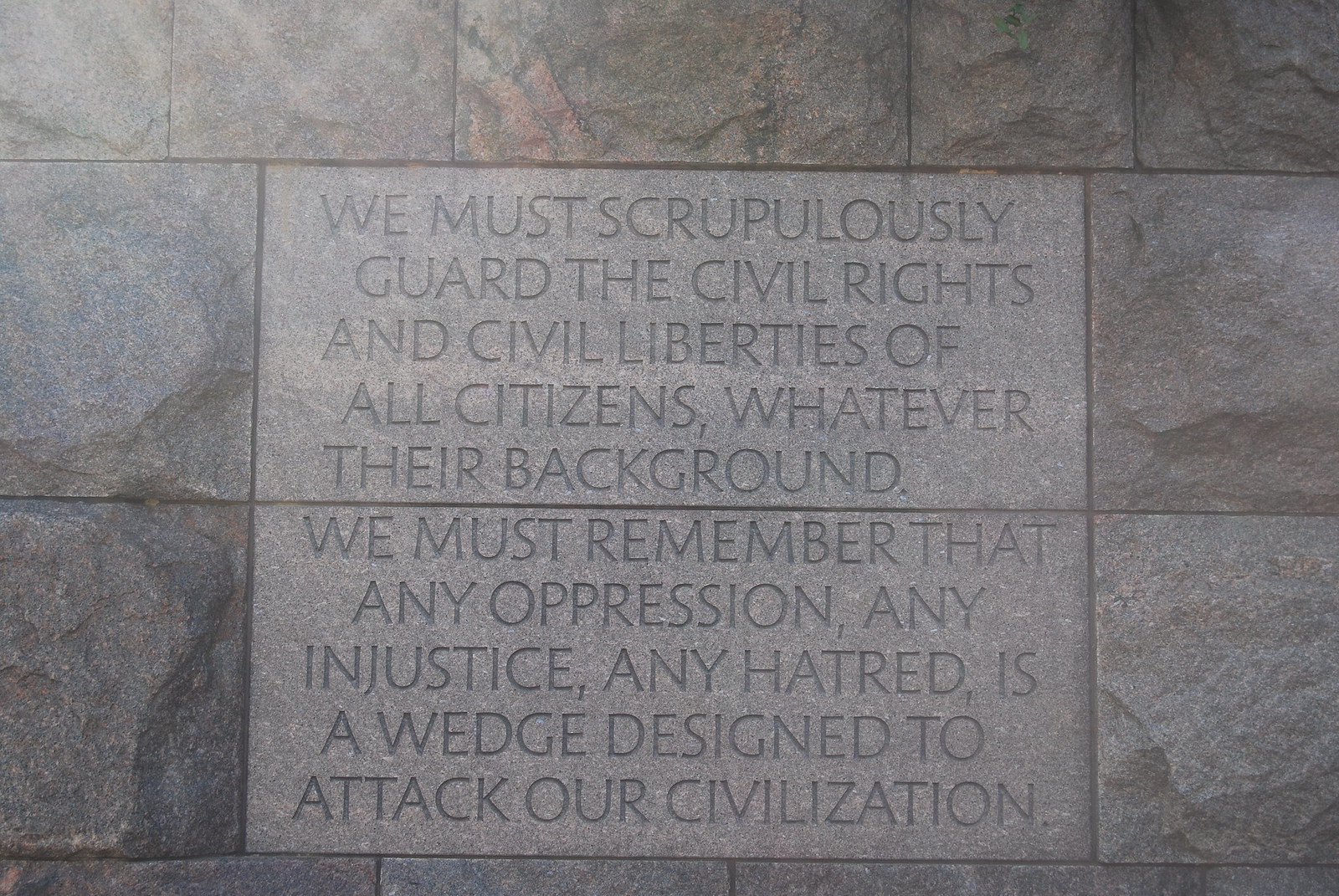The photograph captures a detailed view of a wall or memorial monument composed of large, square stone bricks, predominantly gray with subtle hues of pink and black. The stones, possibly granite or marble, create a striking mosaic of muted tones. At the center, two horizontal rectangular plaques are seamlessly integrated into the wall, featuring a powerful message in professional, all-capital black lettering carved into the stone. The upper plaque states, "WE MUST SCRUPULOUSLY GUARD THE CIVIL RIGHTS AND CIVIL LIBERTIES OF ALL CITIZENS WHATEVER THEIR BACKGROUND," while the lower plaque reads, "WE MUST REMEMBER THAT ANY OPPRESSION, ANY INJUSTICE, ANY HATRED IS A WEDGE DESIGNED TO ATTACK OUR CIVILIZATION." The inscriptions cover three-quarters of the image, giving the impression of a significant and solemn dedication, though it's unclear whether this scene is indoors or outdoors.